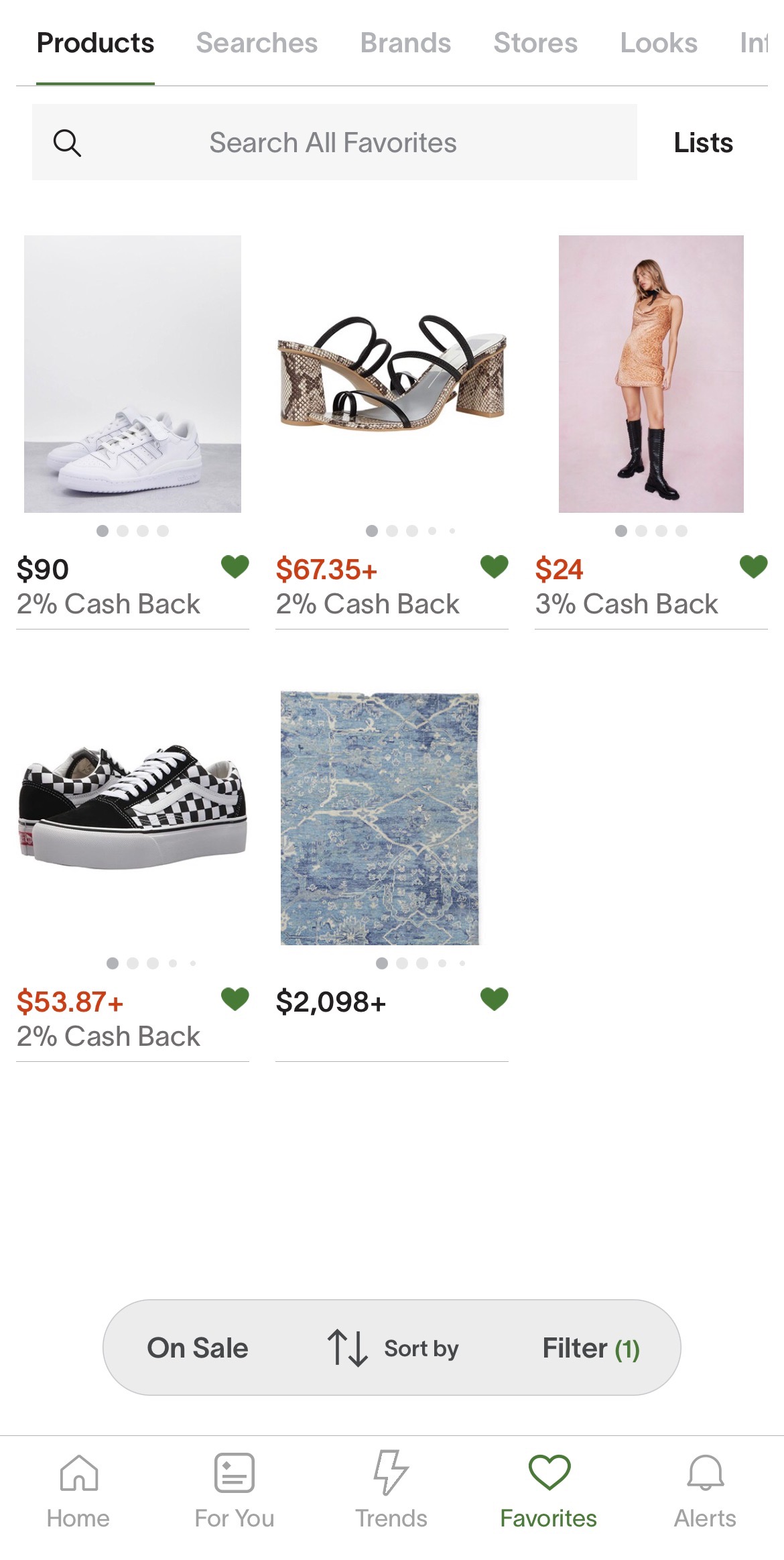A detailed screenshot in portrait mode displays a vibrant, color-rich webpage from a mobile device, likely a smartphone. It is a website dedicated to selling shoes and other fashion-related products. The top navigation bar includes several tabs labeled 'Products', 'Search', 'Brands', 'Stores', and 'Looks', with an additional tab on the far right starting with "IM", though it is partially obscured. Beneath the navigation bar, there is a search bar for entering text queries.

The main content of the display features a selection of products available for purchase. Prominently visible is a pair of sleek white sneakers priced at $90, with an offer of 2% cash back. Users can flip through multiple images of the sneakers, but currently only the first image is shown. Adjacent to the sneakers is a pair of stylish platform shoes for women, priced at $67.35, also offering 2% cash back. Further to the right is a pair of tall black boots modeled by an individual, available for $24. Other products are also viewable, showcasing a diverse range of footwear options.